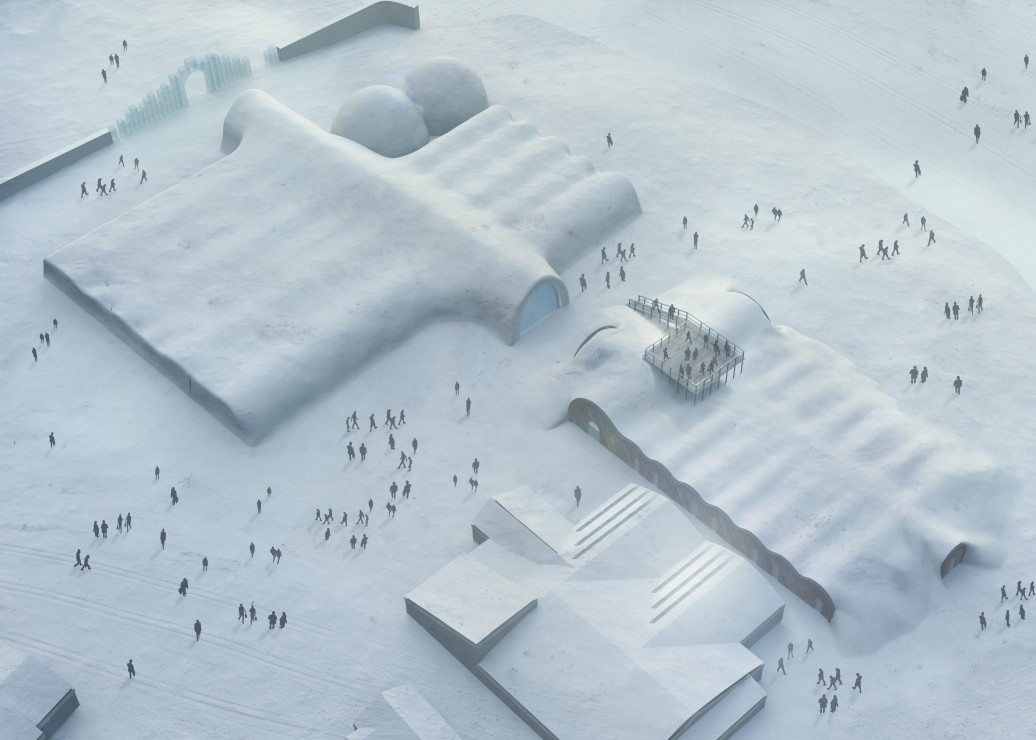This detailed aerial illustration depicts a snow-covered military base in winter, showcasing a network of buildings and bustling human activity. The structures, with their diverse architectural designs featuring both circular and conventional square rooftop layouts, are blanketed by thick layers of snow. In the upper left corner, a snow-covered wooden gate marks the entry point to the base. The central and right sections of the base are particularly active, with numerous small, dark figures navigating the snowy terrain and moving among the buildings. These individuals, who stand out starkly against the pristine white landscape, are scattered throughout the compound. Some are traversing the walkway on the right building, while others are dispersed around the lower left area, midsection, and bottom right quadrant of the image, adding life and movement to this wintry scene.